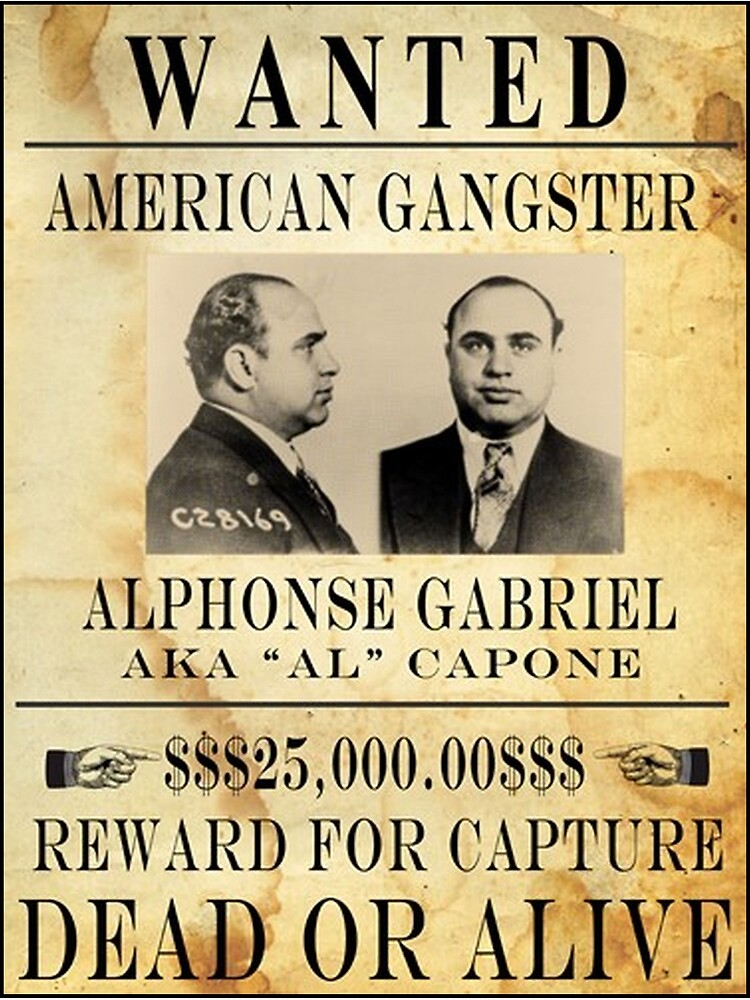The image depicts a stylized, digitally recreated Wanted poster with a thin black border around a sheet of yellowish-brown paper, mimicking an old, stained look but appearing too smooth to be authentic. At the top of the poster, bold black text reads "WANTED," followed by a black dividing line. Below, it states "American Gangster" in non-bold black text. The center of the poster features two mugshots of Al Capone: one profile view showing his right cheek and one frontal view. Capone is dressed in a suit, with short, dark hair, and a round, pudgy face. A number, "C28169," is chalked onto the photographs. Beneath the images, the poster identifies him as "Alphonse Gabriel, aka 'Al' Capone" with another black dividing line below this text. Flanking the reward amount of "$25,000" are small illustrated hands pointing inward, accompanied by money symbols on either side. The phrase "Reward for capture, dead or alive" is below, with "dead or alive" slightly larger and slightly bold.